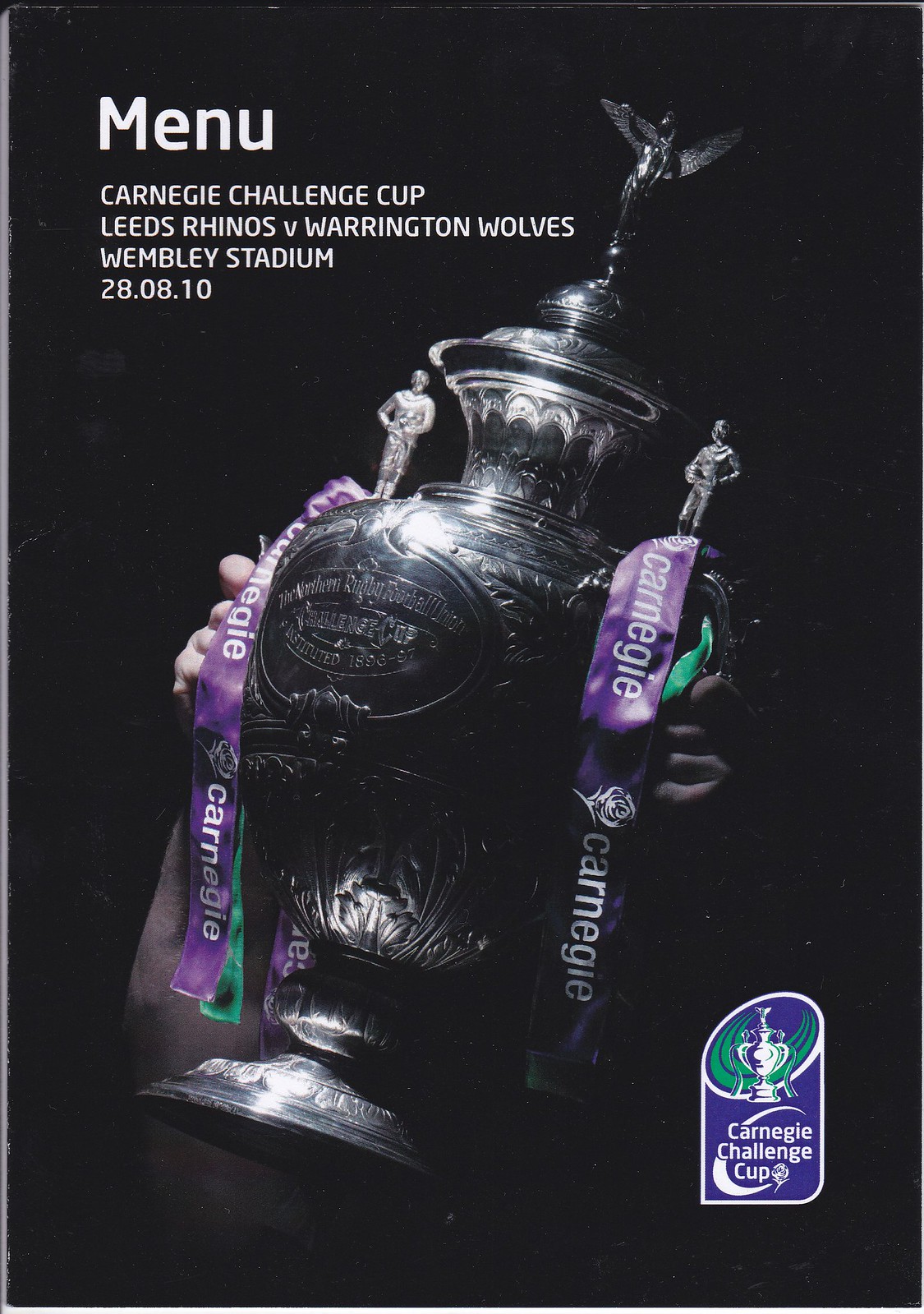The image showcases a prominently featured trophy cup, the Carnegie Challenge Cup, held at an angle that stretches from the lower left to the upper right. Two Caucasian hands grip the handles on either side of the trophy, which is adorned with purple ribbons that display the word "Carnegie." The cup appears to be made of silver or pewter and is depicted with high contrast against a completely black background, making it stand out almost as if it is floating midair. 

Above the trophy, in large white bold text, the word "Menu" is visible. Below this, additional text indicates the event details: "Carnegie Challenge Cup," followed by "Leeds Rhinos vs. Warrington Wolves," "Wembley Stadium," and the date "28th August 2010." The trophy itself has intricate inscriptions, though they are too small to decipher, and features decorative elements including a small angelic figure at the top and smaller figures above the handles. The bottom right corner of the image contains a simplified white outline drawing of the cup alongside the text "Carnegie Challenge Cup" and a logo in green, blue, and white.